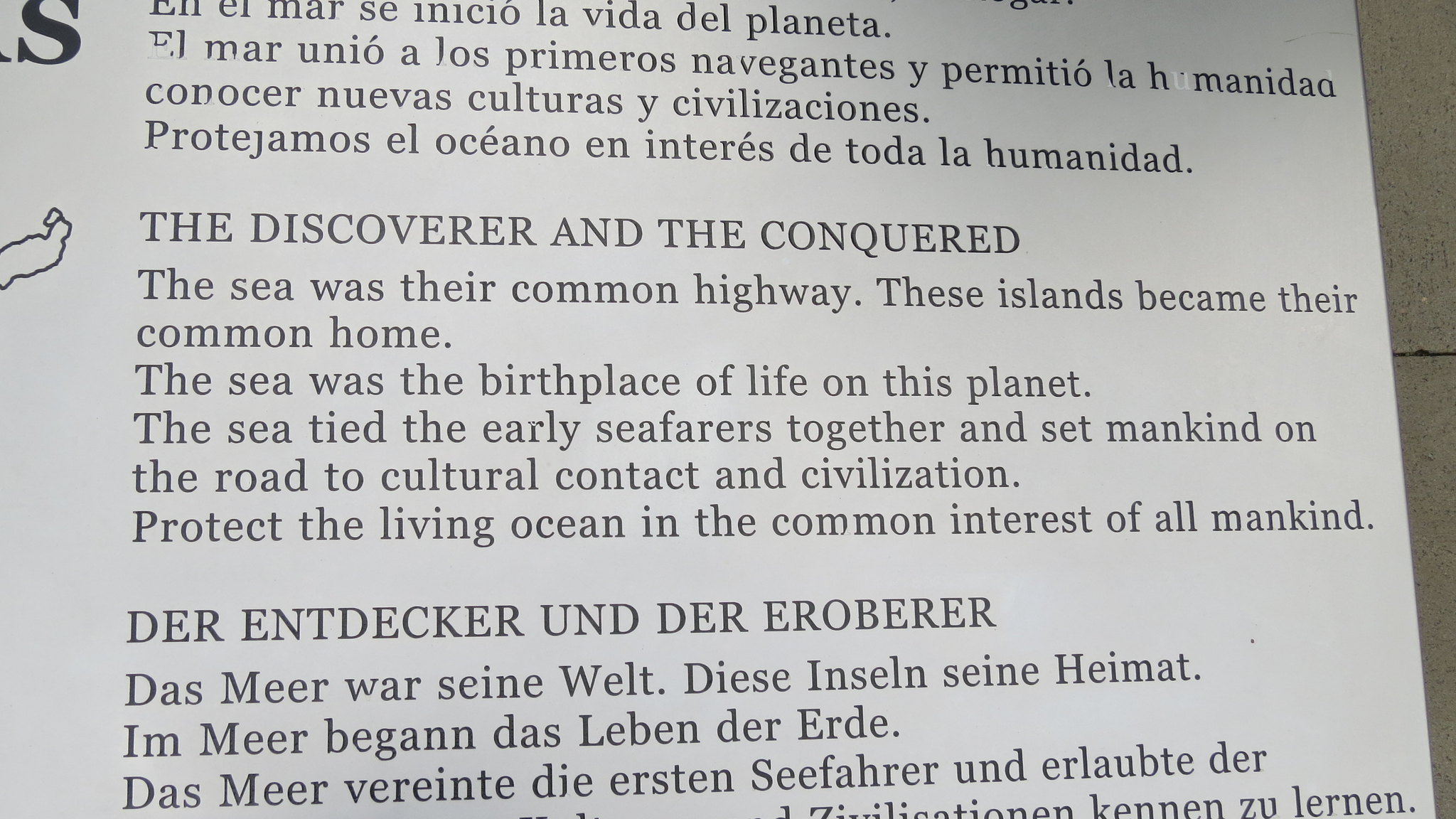The image depicts an informational white placard displaying text in three languages: Spanish at the top, English in the middle, and German at the bottom. The placard is set against what appears to be a granite tile wall or floor. Along the left side, partially cut off, there seems to be an illustration of an island or a map. The English section reads, "The Discoverer and The Conquered," followed by a poetic paragraph: "The sea was their common highway. These islands became their common home. The sea was the birthplace of life on this planet. The sea tied the early seafarers together and set mankind on the road to cultural contact and civilization. Protect the living ocean and the common interest of all mankind." The placard's text, written in black, emphasizes the interconnectedness of humanity through the ocean and calls for the protection of marine life.